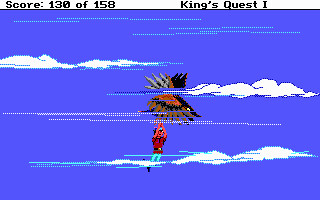In this image, there is a screenshot from an older style video game, reminiscent of classic titles like Galaga or the original Pac-Man. At the very top of the screen, the player’s score is displayed in black, reading "103" or "130" and possibly "158". Below the score, the title "King's Quest I" is prominently featured, with both the "K" and "Q" capitalized and also in black text.

The game's visuals exemplify digitalized, old-school graphics. The background showcases a sky with three distinct, pixelated clouds. Above these clouds, there are a few lines that could represent a horizon or additional elements of the sky. In the center of the screen, amidst the clouds, there is a figure. This character is depicted with a red upper body garment and teal blue pants, standing out vividly against the backdrop. The overall scene captures the charming simplicity and nostalgic aesthetic of early video games.